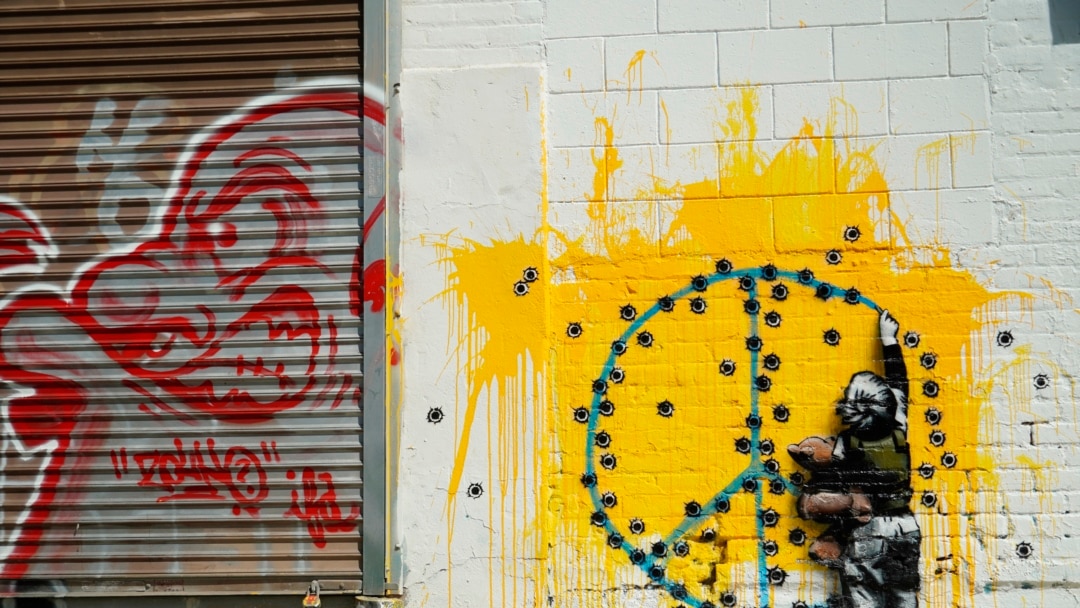This photograph captures an intricate piece of anti-war graffiti art, evocative of the enigmatic street artist Banksy. On the right, a white painted brick and cinderblock wall serves as the canvas. Dominating this wall is a large, central splash of yellow paint, surrounded by drips indicating hasty and deliberate application. Superimposed on this chaotic background is a poignant image of a young boy with short black hair, clad in a green vest and baggy pants. The boy is depicted drawing a large blue peace sign with a crayon or ink, his left arm clutching a teddy bear tightly. This peace sign is marred by numerous bullet holes, arranged almost in the shape of the symbol itself, juxtaposing the innocence of the child's act with stark violence. To the left, another element of the mural features what appears to be a grimacing face, possibly of a bald man with an exaggerated chin, painted in red on a grayish-white roll-up door, adding an additional layer of intensity to the scene. The stark contrast in themes and colors effectively underscores the powerful anti-war message.